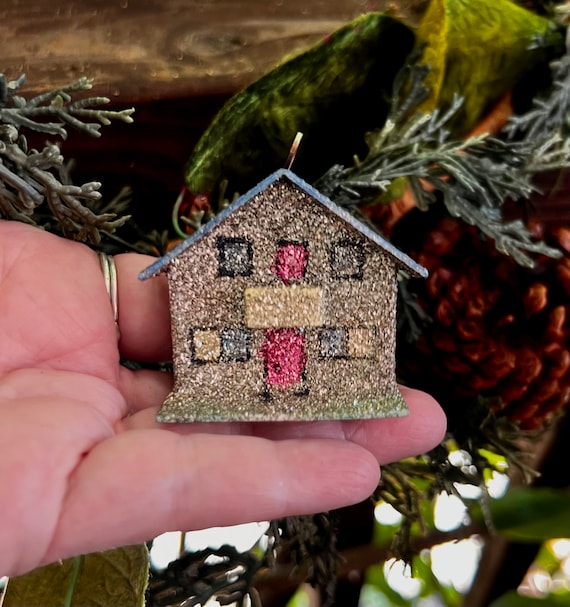In this close-up image, we see a person's hand, adorned with a silver ring on the index finger, holding a tiny ornament shaped like a house, reminiscent of a gingerbread house but likely made from stone and covered in gold glitter. The miniature house, which is smaller than the person's little finger, features a glittering blue roof with a hook on top. The front of the house is detailed with painted windows in alternating colors: black, red, and tan, along with a red front door and green glitter-covered grass at the base. The background hints at a festive setting, possibly a Christmas tree or wreath, with visible elements including a brown pine cone, green leaves, and a strip of wood.